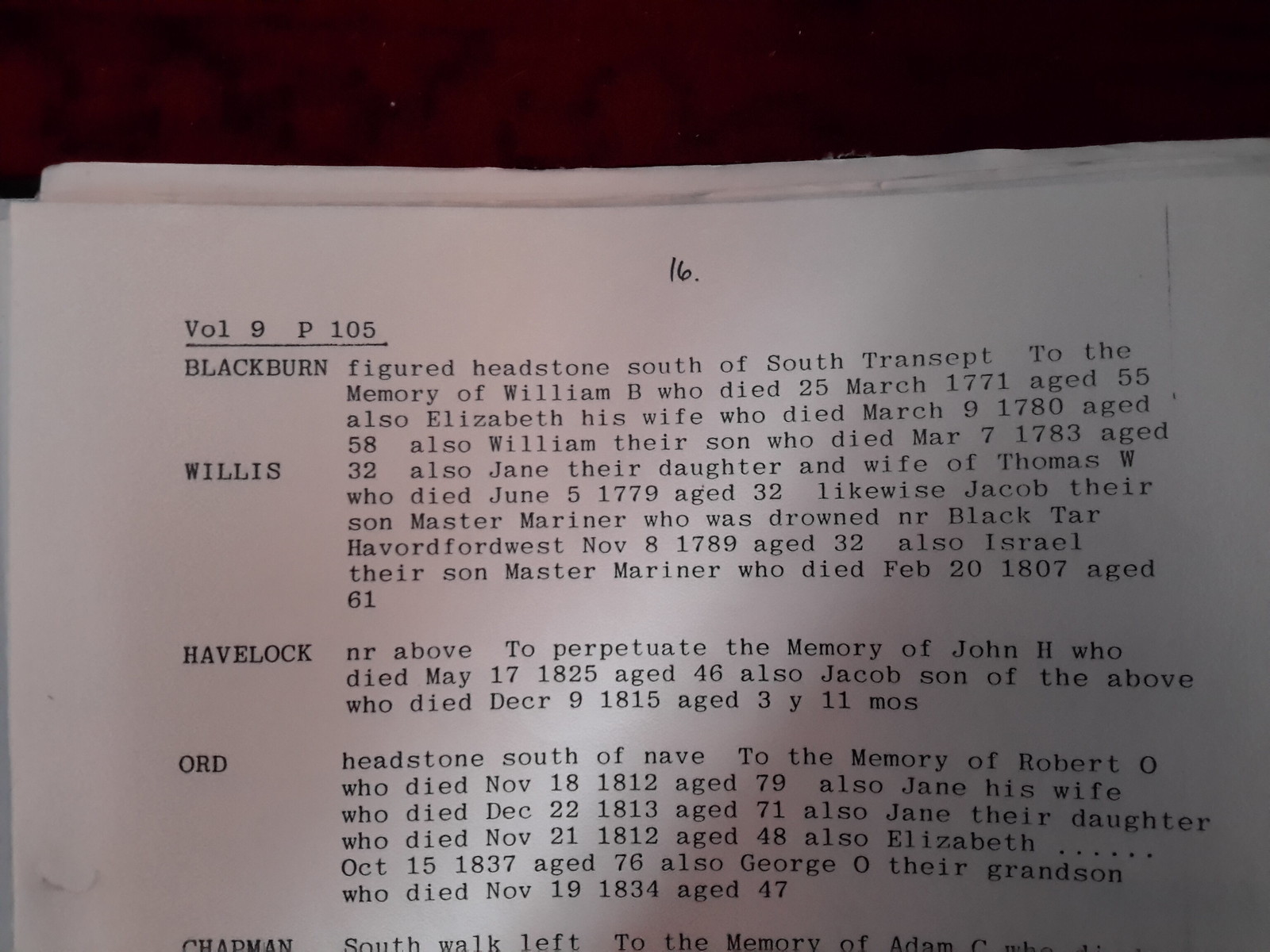This is a photograph of a typewritten page from a book or pamphlet, exhibiting the top half of the page along with the edges of two or more pages slightly visible at the top. The page is white with black typewritten text and features a handwritten number "16." Below this number, an underlined heading reads "Volume 9, P. 105." In the left-hand column, a list of names is presented in uppercase type: "BLACKBURN," "WILLIS," "HAVELOCK," "ORD," and "CHAPMAN." Adjacent to these names are detailed descriptions of and locations for headstones, with information quoted directly from the headstones. For instance, next to "HAVELOCK," it reads, "NR above to perpetuate a memory of John H. who died May 17, 1825, age 46. Also, Jacob, son of the above, who died December 9, 1815, age 3 years, 11 months." Similarly, beside "BLACKBURN," it states, "Figured headstone south of South Transept, to the memory of William B, who died 25 March 1771, age 55." The top part of the photograph shows a black section with some hazy, splotchy red areas spread across the left to the center.